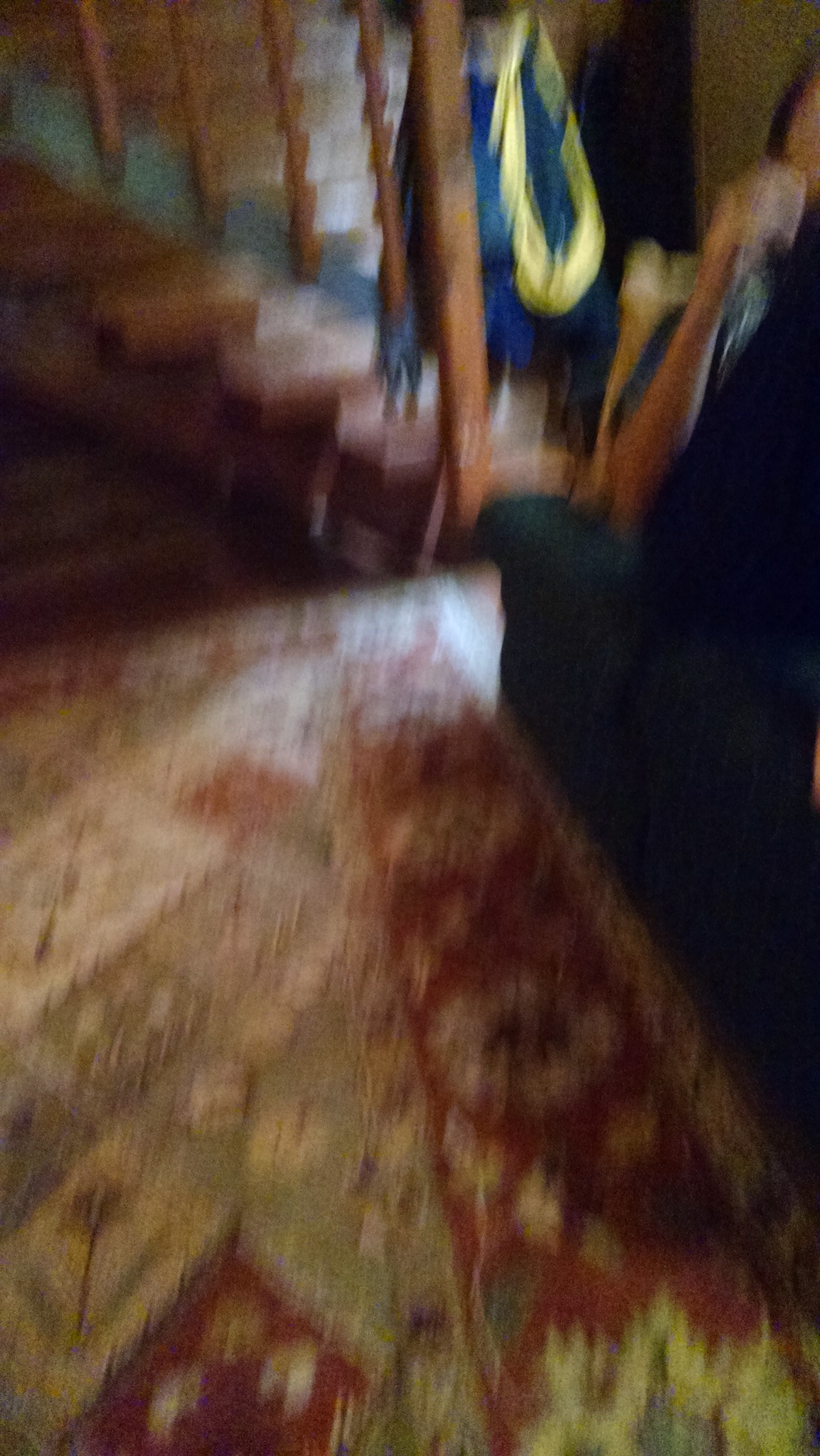In the image, there is a cozy living room featuring a wooden floor adorned with an area rug. A blue couch is prominently situated in the scene, and off in the distance, there's a stairwell. Seated on the couch is a man wearing a light blue, short-sleeved shirt and dark blue pants. His attire reveals his arm and hand, and half of his face is visible. He has short black hair, although it's partially cut off in the image, suggesting it could be styled into a ponytail, but it's more likely a short haircut. The stairwell in the background has a coat hanging on one of the rails, possibly a blue puffer coat with a yellow-trimmed scarf, though the image is slightly blurry and details are hard to discern.